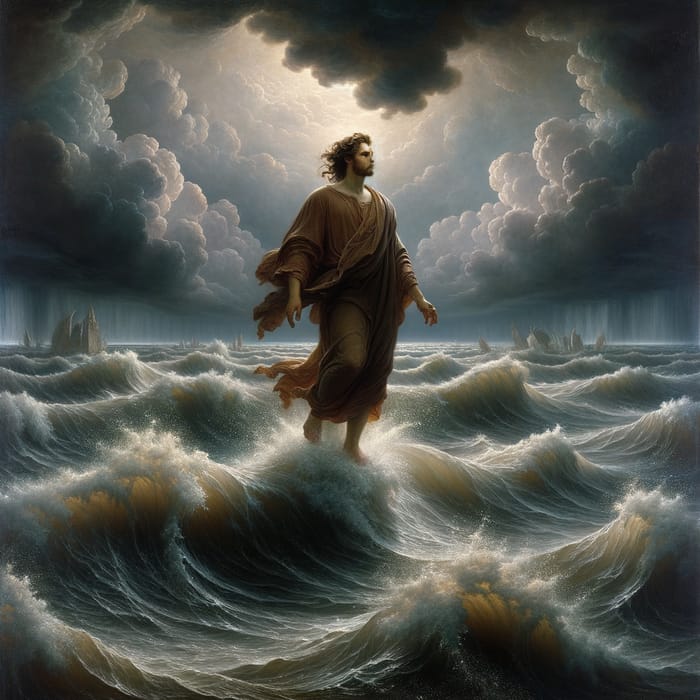This image is a square painting, approximately five inches high by five inches wide, depicting an intensely stormy seascape. The lower half showcases high, turbulent waves in murky brown tones with amber tips and dark white crests. At the center of this churning sea, a man, presumed to be Jesus, strides atop the waves. He has fair skin, long, wavy brown hair blowing backward in the wind, and a mustache and beard. Clad in a flowing brown robe and barefooted, he faces slightly to the right. The background reveals what could be ruins or rocks jutting out of the water.

The sky above is moody and evocative, filled with thick, dark gray clouds arranged in circular patterns that lighten towards the center. A stark black cloud descends along the middle, forming a heart-like shape with lighter clouds radiating from its center. This central light gently illuminates the stormy scene below, enhancing the drama and mystique of the painting.